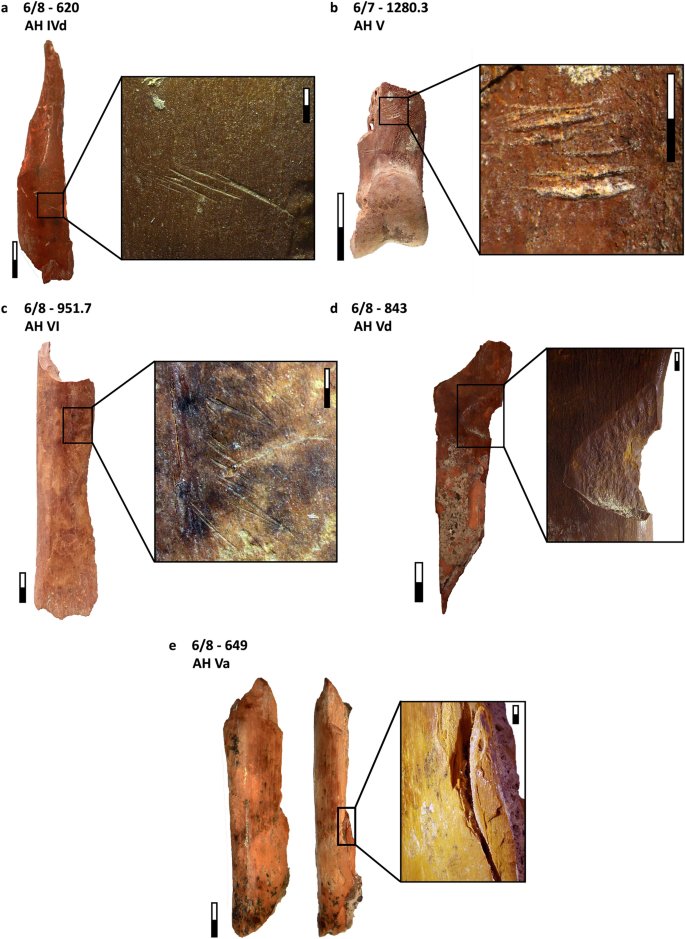The image features six long, narrow artifacts, primarily dark red to light pinkish in color, meticulously presented with a dual photograph layout. Each artifact on the left side is accompanied by a highly magnified close-up on the right, linked by arrows pointing to specific portions of the artifacts. The artifacts are uniformly upright and appear to vary subtly in specific shapes and sizes but are generally consistent in length. Detailed labels accompany each artifact, such as A6H-620AHIVD, B67-1280.3 (AH B), and C6H-951.7 (AH VI), signifying their unique identifiers. The zoomed-in images reveal intricate details and color variations within the artifacts, although they are primarily shades of brown, hinting at their possible material composition, likely bone or stone fragments.